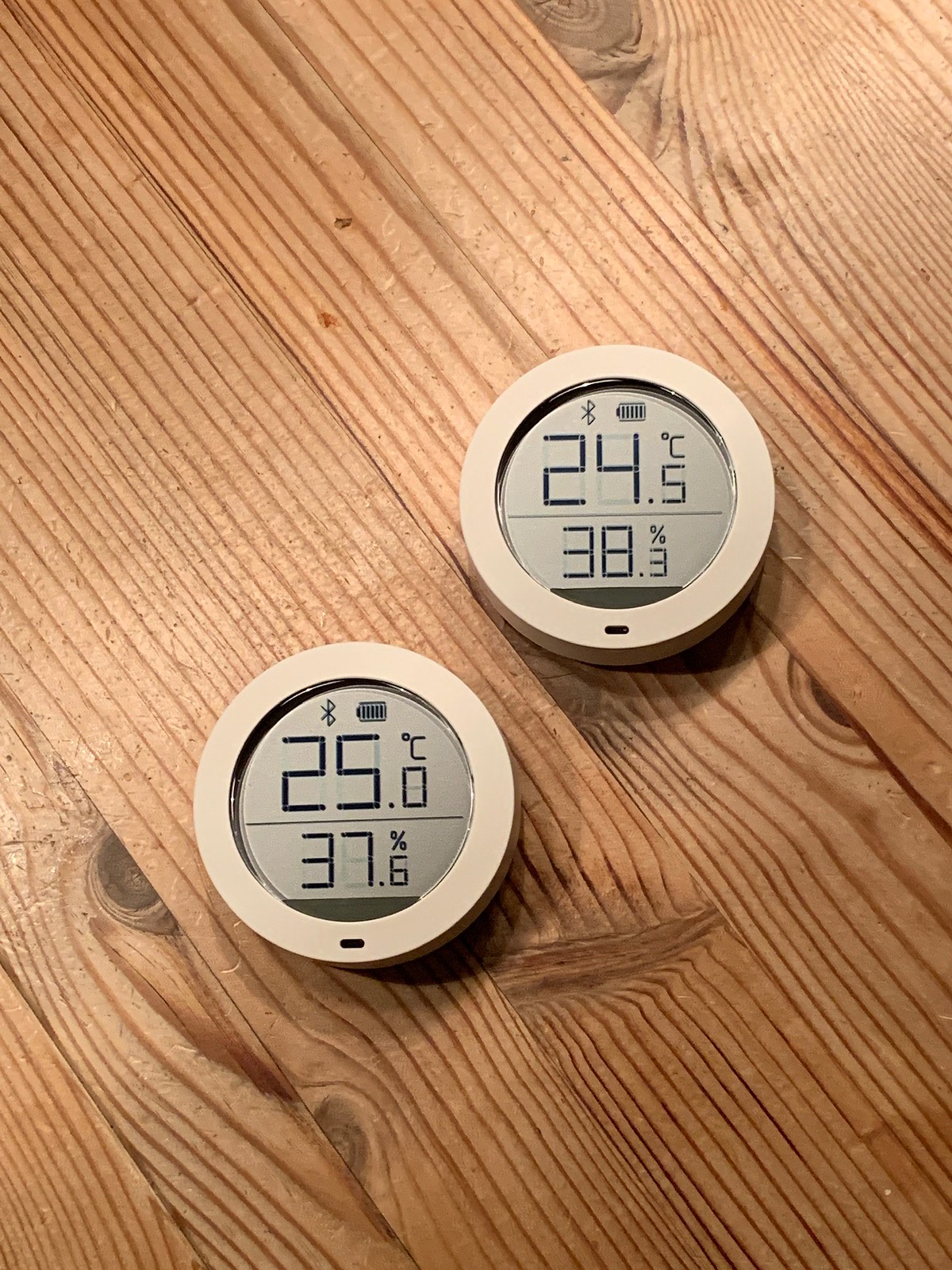This overhead photograph captures two identical circular electronic devices placed on a rustic wooden surface composed of several boards, their grain running diagonally from the upper left to the lower right. The wood features distinct knots along the board edges, adding texture to the setting. The exact nature of the wooden surface is ambiguous—it could be a floor, table, or shelf.

The two devices, resembling discs or pucks, are centrally positioned with the upper one being closer to the right edge of the frame. Each device has a digital display and features a Bluetooth icon and a fully charged battery icon at the top of their screens.

The upper disc displays a temperature reading of 24.5 degrees Celsius and a humidity level of 38.3 percent beneath that. The lower disc shows a slightly higher temperature of 25.0 degrees Celsius and a humidity level of 37.6 percent. Both devices also have small ovals at their bottom edge, indicative of USB-C charging ports, suggesting they are rechargeable. The precise craftsmanship of the wooden surface, combined with the modernity of the electronic discs, makes for an intriguing composition.